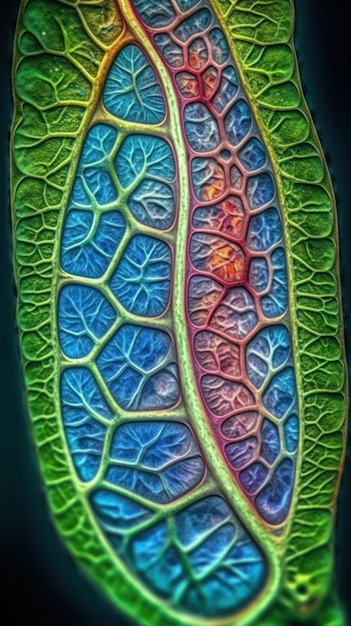This close-up image, taken under a microscope, showcases a cross-section of a leaf that appears to have been dyed to highlight its intricate structure. The photograph vividly presents the outer edges of the leaf in their natural green color, indicative of chlorophyll presence. Progressing inward, the veins become the focal point, especially the prominent central vein, which is strikingly blue. Adjacent to the central vein on the right, the leaf displays a gradient of dark red and purple hues, blending back into blue farther from the center. The varying colors may represent differences in oxygen flow or other liquids within the leaf. The detailed image also reveals individual cells and an array of smaller veins branching out from the larger ones. There are no annotations or text included with this photo.